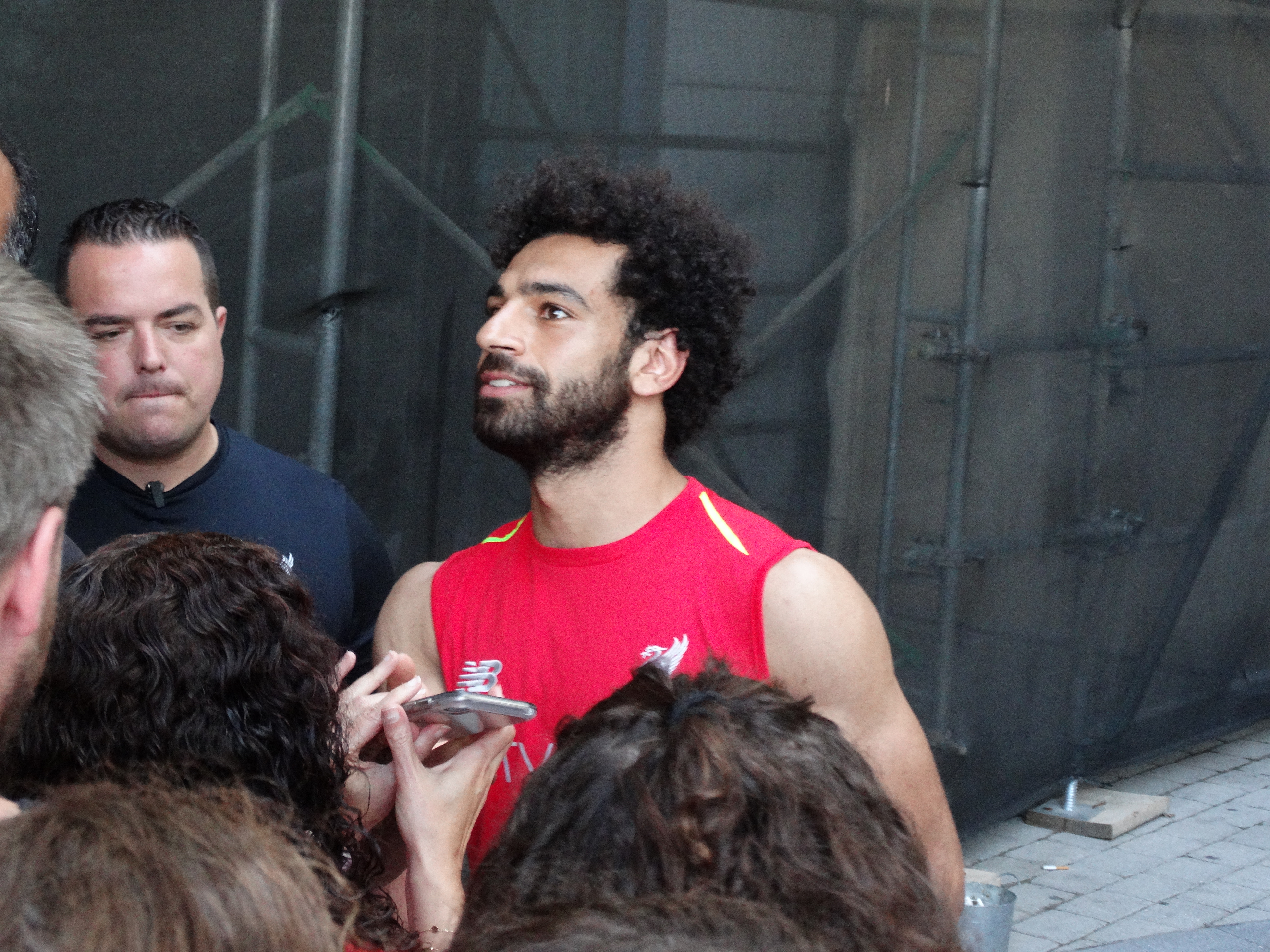The photograph captures a dynamic interview scene set against a construction area outdoors, presumably in the middle of the day. Centered in the image is a muscled man with a bearded face and black, short, curly hair. He is clad in a sleeveless red shirt with distinctive yellow stripes on the shoulders and a partially obscured white NB logo on the chest. His engaged smile is directed towards the five individuals facing him with their backs to the camera. One person among them is prominently holding up a silver smartphone towards him, evidently recording or taking a photo. To the man's left, another individual wearing a blue shirt and a lapel microphone on their collar is captured gazing downward pensively, contributing to the scene's sense of focused attention. The setting highlights a variety of background elements, including a stone surface underfoot and a mesh wall with metal poles in the distance, adding to the overall vibrant and busy atmosphere. The colors in the image span different shades of gray, red, tan, brown, black, and pink, enhancing the visual complexity of the event.